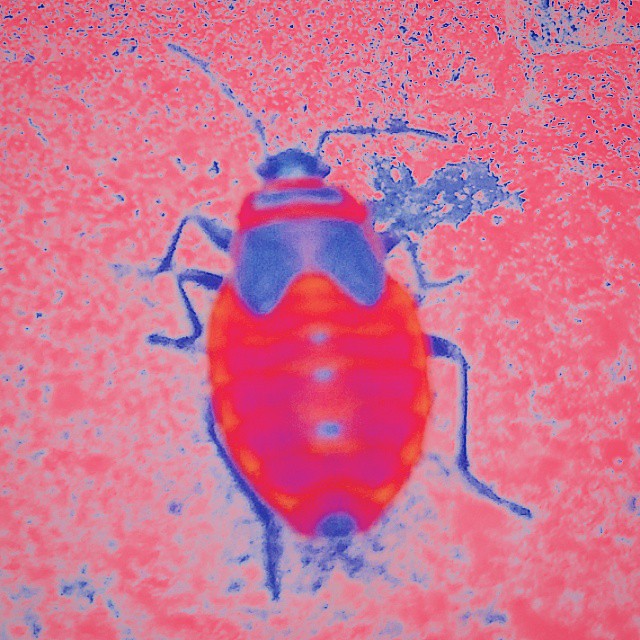The image features a modern abstract painting of a bug, captured from above, with a distinctive color scheme dominated by red, blue, and hints of pink and purple. The background is a mix of pinks, purples, blues, and some gray, creating a patchy, splattered effect. The bug itself has a bulbous, reddish-pink body that is smaller at the top and larger at the back, resembling the shape of a tick. Its midsection is blue, transitioning to a blue head adorned with two large antennas—one bent to the right and the other almost straight up. The bug has six thin, bent blue legs, suggesting it’s standing on a surface. There are also several white spots on its body, likely indicating light reflections. The overall appearance of the image is distorted, giving the impression that it may be viewed through a filter or under a microscope.